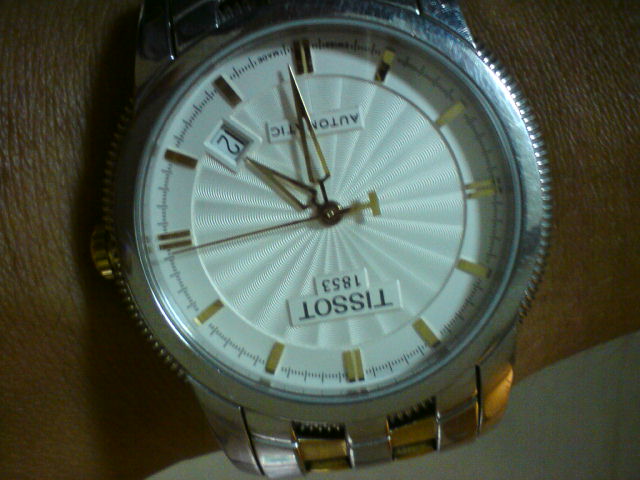The image features a Tissot watch with a prominent silver face, encased in a bezel that has a textured edge. The watch's face displays the brand name "Tissot" in large letters, with the year "1835" noted below it. Surrounding the face are finely detailed hash marks indicating the minutes. At the top of the watch face, the number "2" is visible, suggesting it's part of a date window or additional feature. The watch is paired with a sophisticated brown leather strap, accented by a section of white material at the bottom right. There's a dial on the left side of the watch, possibly for adjusting the time or date. The bottom of the watch indicates silver hinges, which show signs of wear with visible scratch marks, adding a touch of character to the timepiece.